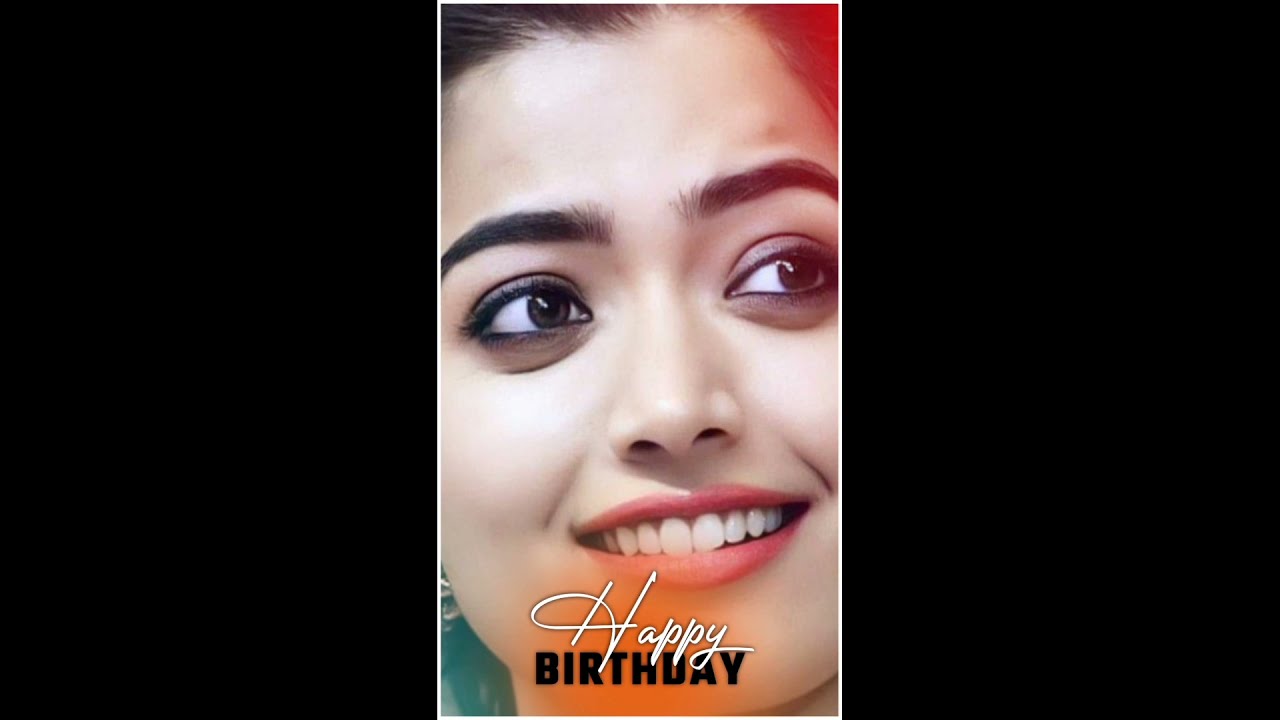The photo depicts a young woman, likely in her mid to late 20s, with dark hair pulled back, accentuated by a generous application of makeup, including significant dark shading under her expressive brown eyes. She wears a broad, joyful smile that reveals her teeth as she looks slightly upward and to her left, away from the camera. A bold caption at the bottom corner reads "Happy Birthday," with "Happy" in a large, sweeping off-white cursive font and "Birthday" in thick black block letters, all encased in a neon-like pattern with a white border.